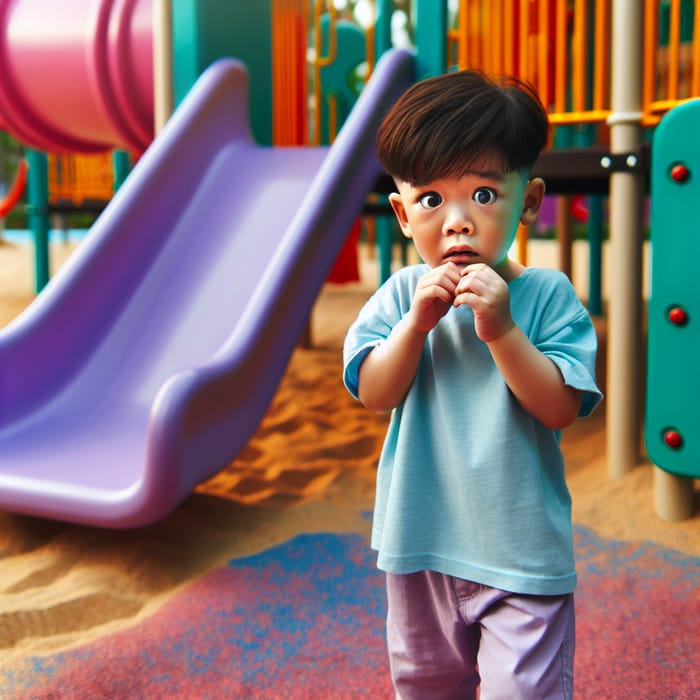A highly detailed and realistic image, giving the appearance of cartoonish, computer-generated artwork, showcases a young boy, possibly of Asian descent, around 3 to 5 years old, standing on a playground. His big, wide, brown eyes, exhibiting a terrified and worried expression, are emphasized by his short brown hair. He stands with his hands clasped just below his mouth, dressed in a short-sleeved blue shirt and purple shorts, amidst colorful playground equipment including a prominent purple slide directly behind him, orange bars, and various structures of green, yellow, pink, cyan, and purple hues. The playground surface beneath him and around is a mix of regular sand and patches of blue sand, creating a vibrant but slightly unsettling scene under daylight.